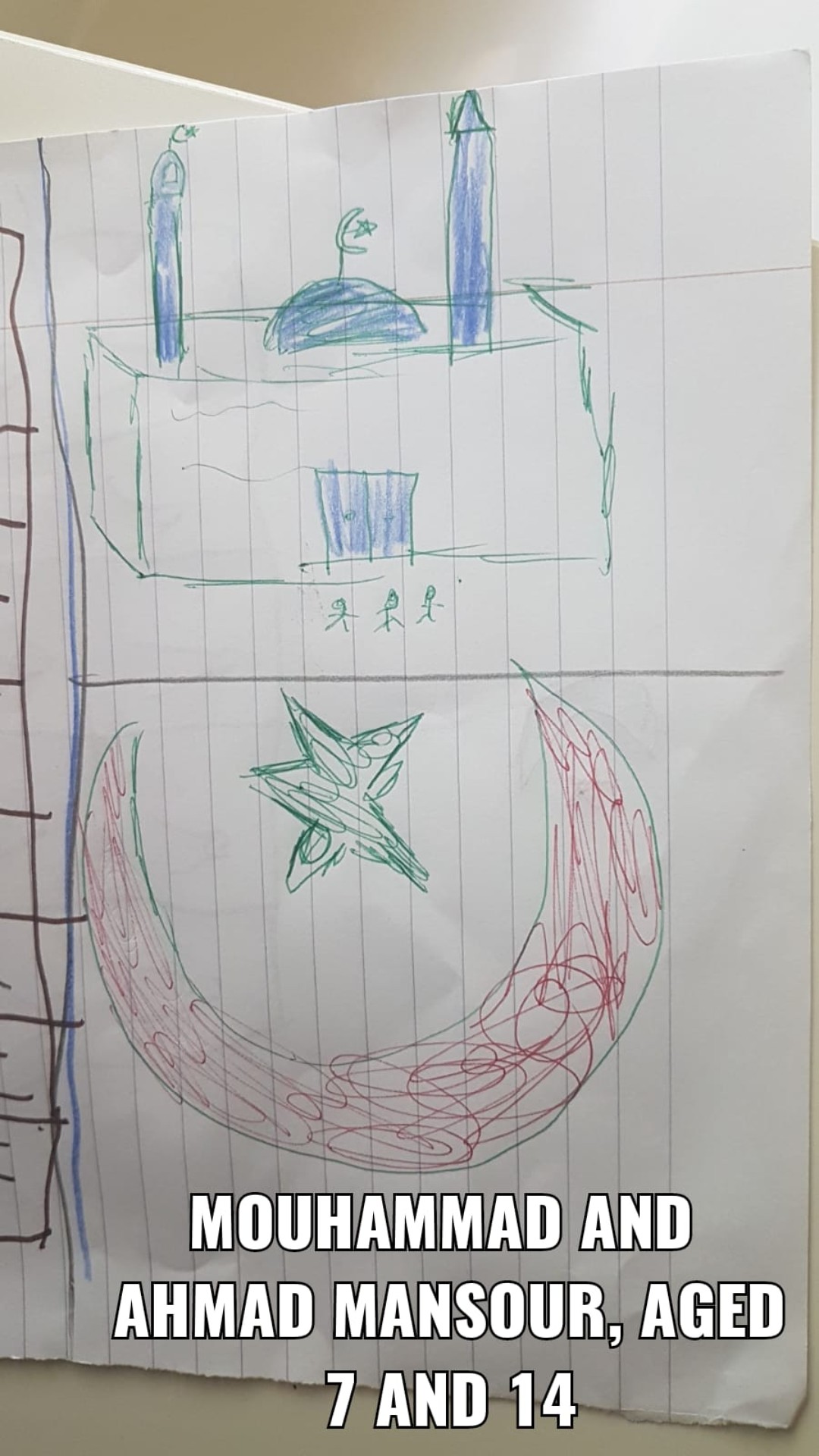The image depicts a child's drawing on a piece of notebook paper oriented horizontally, with the left side facing upward. The notebook paper features the characteristic holes along one margin, indicating it has been turned sideways. The drawing itself is divided by a faint gray line across the upper portion. 

In the lower part of the drawing, a crescent moon is prominently showcased in a playful, imaginative style. Adjacent to the moon is a star, colored in a vibrant green hue.

Above the gray dividing line, a simple representation of a house is illustrated. The house is cube-shaped with a blue door situated in the middle of its facade. Two cylindrical structures protrude from the top of the house, adding an element of whimsy to the child’s depiction.

The entire artwork exudes a sense of innocence and creativity, capturing the youthful essence of the artist.